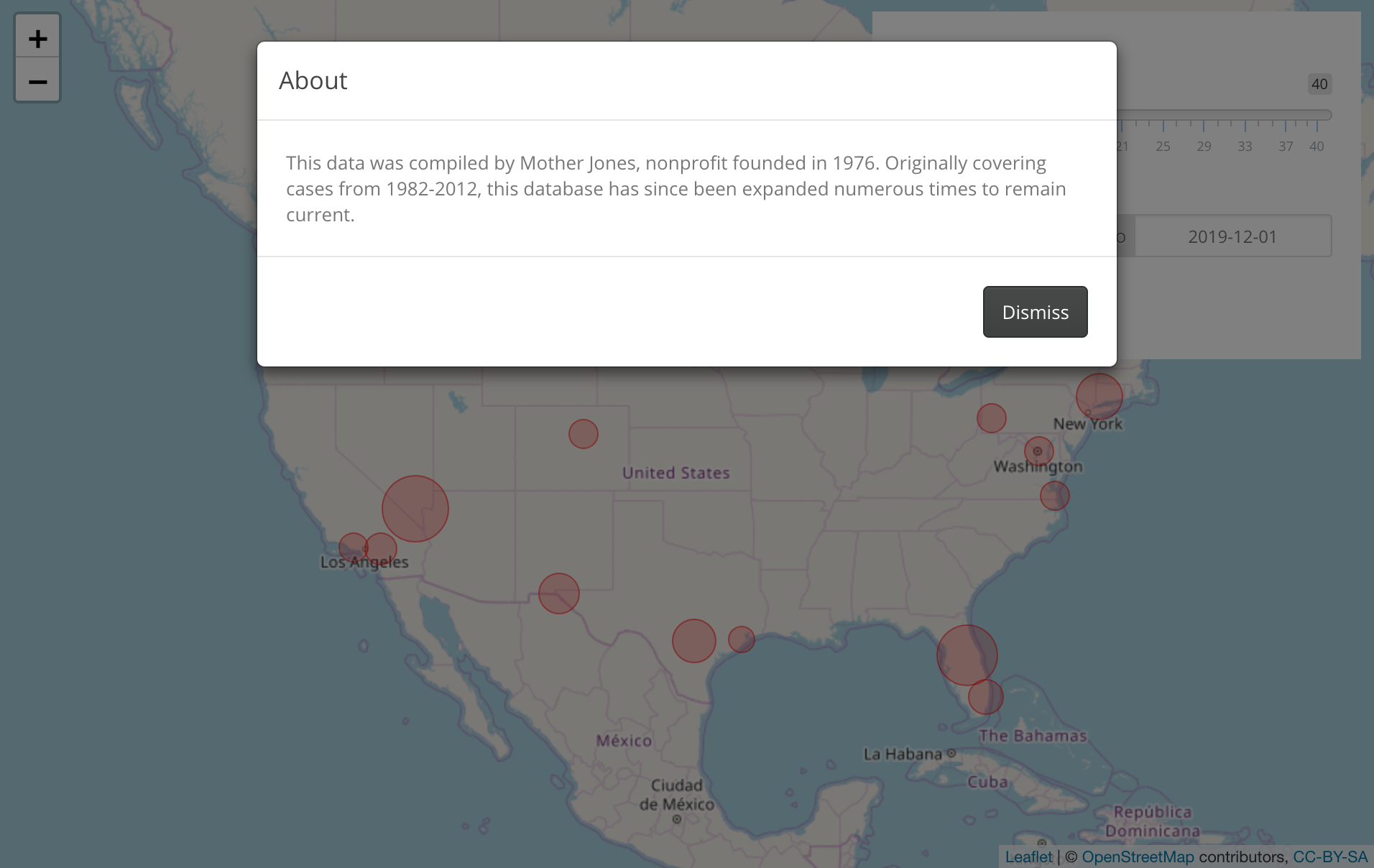The image showcases a map of the United States as the background, which is grayed out to highlight a pop-up box. Despite the gray overlay, the map still reveals the oceans in a grayish-blue hue and the land of the states in a grayish-lavender shade. Scattered across various states are solid pink circles of different sizes, indicating specific locations. Notably, there are a few pink circles in Florida, one in New York, one in Washington D.C., one in the southern part of Virginia, and another near Pittsburgh in Pennsylvania. The state borders are clearly outlined, though state names are not mentioned.

A prominent large pink circle appears where Nevada, Arizona, and California intersect, with a few sizeable circles over Los Angeles. The focal point of the image is a white rectangular pop-up box with gray text. The header reads "About," followed by a description explaining that the data was compiled by Mother Jones, a non-profit organization founded in 1976, initially covering cases from 1982 to 2012 and updated multiple times to remain current. In the lower right corner of the pop-up box is a black rectangular button with the word "Dismiss" in white text.